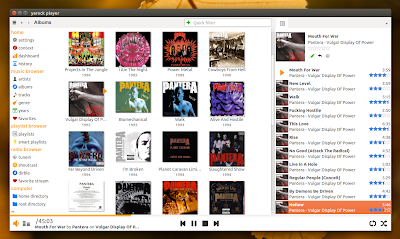This screenshot captures a media player interface on a computer, likely operating on Mac OS, as indicated by the iconic minimize, maximize, and close buttons located in the upper left corner. The interface boasts a clean, white color scheme with vibrant orange accents, enhancing its modern aesthetic. Prominently featured in the center of the screen are various musical albums, with several albums by Pantera taking center stage. To the right, a detailed playlist displays the songs queued for playback, complete with a star rating system ranging from one to five stars, allowing the user to rate each track. Currently, a song is playing and is about one-third of the way through, evident from the progressing orange bar at the bottom of the media player. The application window is positioned centrally on the desktop and is not in a maximized state.